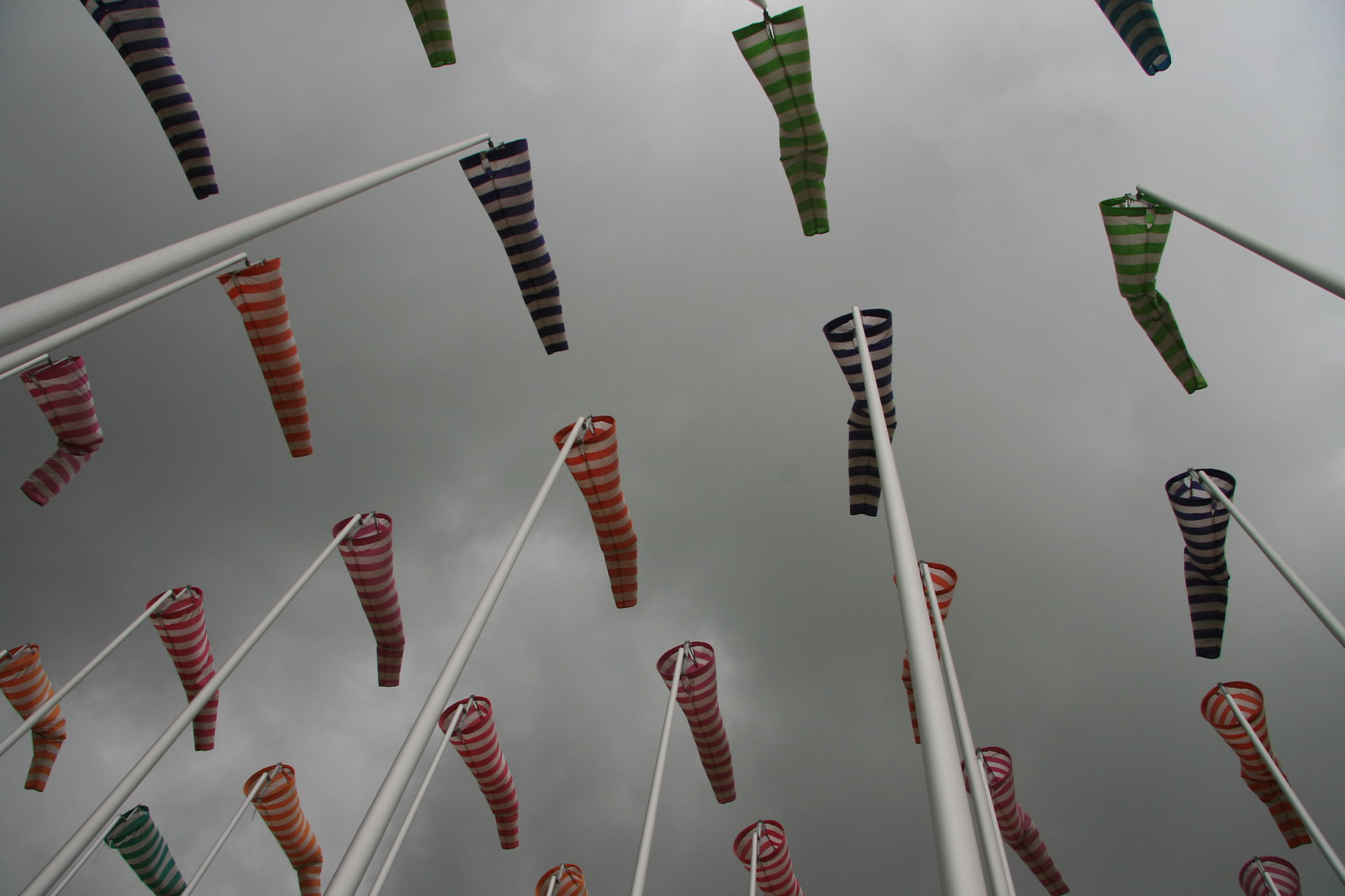This is a color photograph taken during the daytime, capturing a scene from the ground looking up towards the sky. The sky is filled with light gray, very cloudy, dark rain clouds, indicating an impending storm that hasn't yet begun. High above on slender white poles, numerous windsocks fill the frame. These windsocks, which are tapered like funnels or long narrow stockings, come in different colors and striped patterns. The predominant colors are green and white, purple and white, red and white, with a notable number of blue and white striped windsocks as well. The windsocks are arrayed at various angles, creating a dynamic and chaotic visual against the overcast sky.